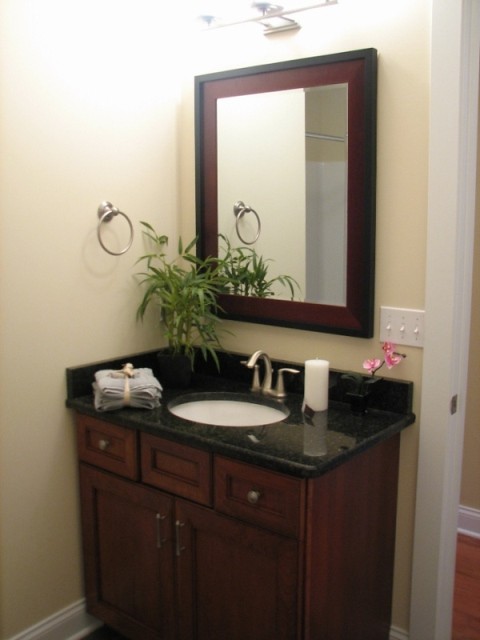The image, in portrait orientation, showcases a meticulously designed bathroom sink area bathed in ample light from an overhead sconce. At the center of the scene is a framed mirror, bordered by a sleek black outer frame with a rich maroon inner matting. Adjacent to the mirror, mounted on the wall, is a towel ring.

The sink rests atop a dark marble countertop, which contrasts elegantly with the brass fixtures comprising a central water spout flanked by hot and cold water levers. Below the countertop, the cabinetry is fashioned from warm brown wood, providing a grounded and earthy feel to the decor.

In the corner of the countertop, a vibrant bamboo plant adds a touch of greenery, while to the right, an orchid plant introduces an exotic floral element. Three light switches are situated just above the orchid, enhancing the functionality and utility of the space.

Accentuating the sink area, a white candle is placed next to the faucets, contributing to an atmosphere of relaxation. Additionally, neatly rolled towels, tied with a ribbon, sit near the sink’s opening, complementing the pristine white interior of the sink. This carefully curated assembly of elements presents a harmonious blend of luxury and nature within the bathroom.